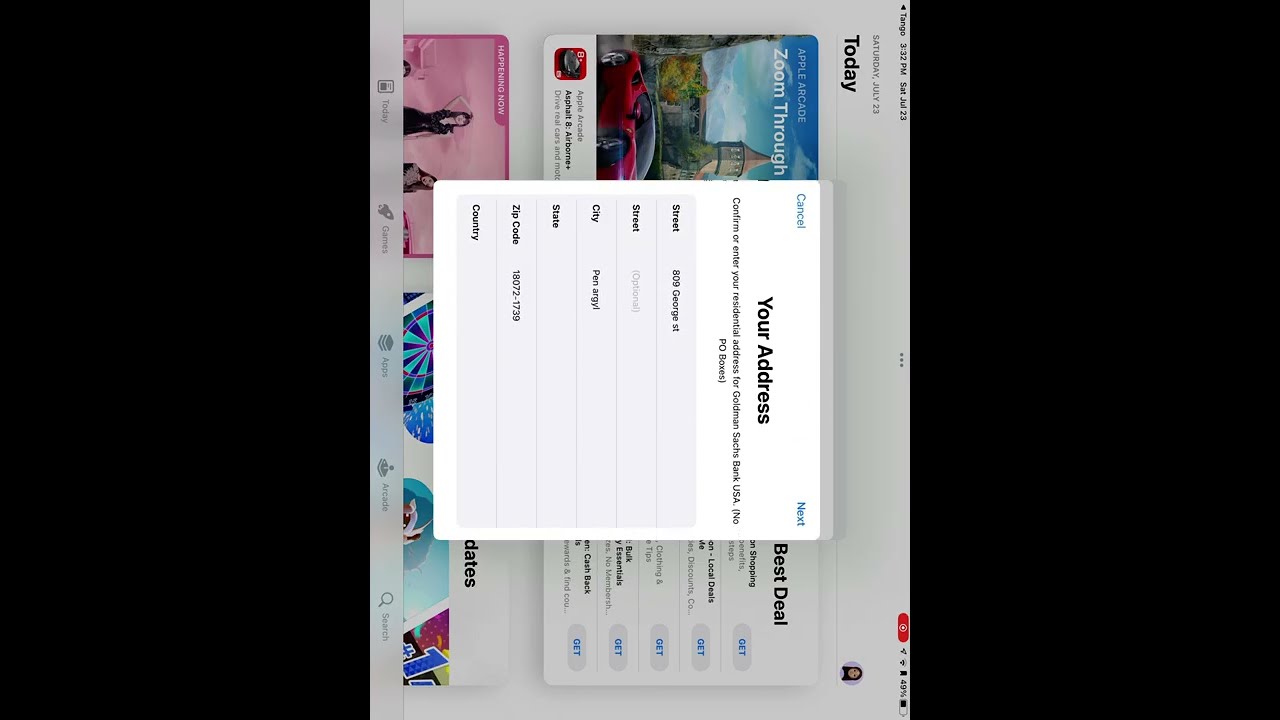The image depicts a horizontally oriented screenshot of a tablet or phone screen, notable for its rotated, 90-degree counter-clockwise display, framed by black bars on the left and right. At the center, a prominent, white pop-up box prompts the user to "Confirm or enter your residential address for Goldman Sachs Bank, USA Inc.," explicitly stating "No P.O. Boxes." The top left corner of this box features a "Cancel" button, while the top right corner displays a "Next" button. The form requires details such as "Street" (filled with "809 George Street"), "City" ("Penn Argyle"), "State," "Zip Code" ("18072"), and "Country."

Behind this primary form, the underlying screen shows additional content. At the top, the date "Saturday, July 23rd" is visible, followed by the phrase "Zoom Through." Further elements include a banner labeled "Best Deals" in the top right corner, as well as a variety of app icons or options beneath it. Specific apps mentioned are "Apple Arcade" and "Asphalt Airborne," along with a visual of a vehicle and building, resembling a castle, set amid trees. There are also sections featuring different colors like pink, blue, green, white, gray, black, yellow, aqua blue, magenta, and red; one notable pink box contains an image of a woman in a black dress. Additionally, a pie-wheel graphic with the number one is seen adjacent to the pink box.